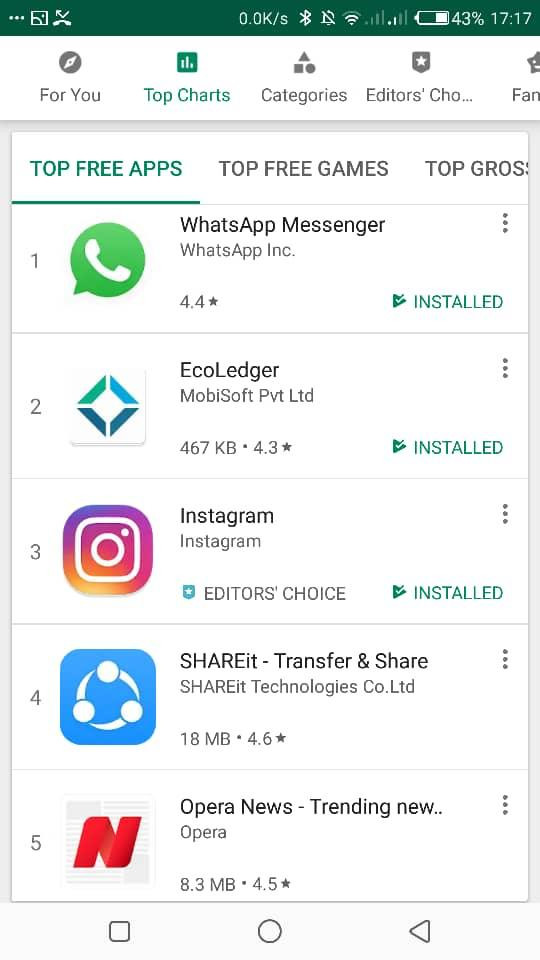Screenshot of a mobile app interface:

The screenshot is a vertical, rectangular image indicative of a mobile phone display. At the top, a green status bar contains various icons and information. On the right side of this bar, the time is displayed as 17:17, next to a battery icon showing 43% charge. Additionally, there are two signal bars and a Bluetooth icon. Towards the center-left section of the bar, there are several other icons, including a set of three dots, indicating a menu, and icons suggesting ongoing call functionalities, such as photo, video, and phone handset symbols.

Beneath the status bar, the background primarily displays a white interface. Across a gray navigation bar are buttons for "For you," "Top charts," "Categories," "Editors' Choice," abbreviated as "CHO," and another option cut off from the view. The "Top charts" button is highlighted in green, indicating it is currently selected.

Below this navigation bar, there is a section titled "Top free apps," suggesting the selected category. It lists the top free apps along with their corresponding icons and names. The apps listed include:
1. **WhatsApp Messenger:** Icon - a green speech bubble with a phone.
2. **Ecolinger:** Icon details are not provided.
3. **Instagram:** Icon - a square with iridescent shades of pink and orange.
4. **Shared:** Icon details are not provided.
5. **Opera News:** Icon details are not provided.

At the very bottom of the screenshot, there are three navigational icons reminiscent of Android's navigation buttons: a square, a circle, and a triangle, likely representing recent apps, home, and back functions, respectively.